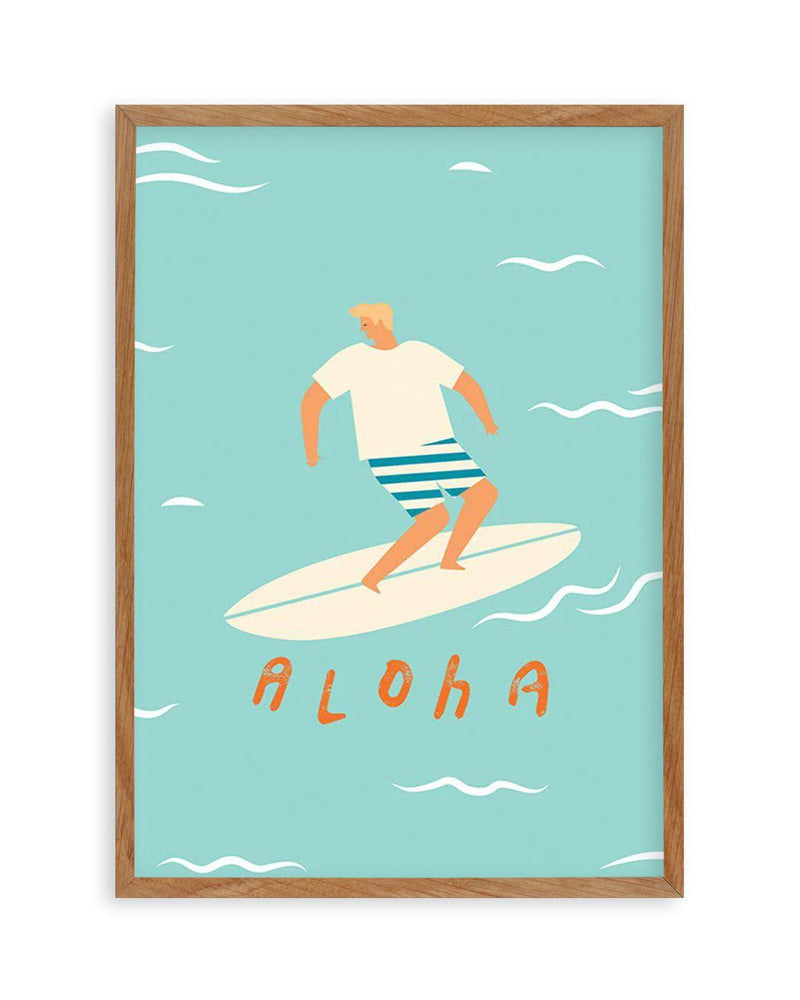This image is a digital art piece showcased within a thin, light-colored wooden frame. It depicts a white male figure with blonde hair surfing on a white surfboard, which features a turquoise stripe running down its center that seamlessly blends with the surrounding ocean water. The man is dressed in a white cotton t-shirt and blue and white striped shorts. The surfboard hovers above water illustrated with white, squiggly lines to indicate waves. Beneath the surfboard, the word "Aloha" is scrawled in a messy, orange marker-like font. The composition is playful and colorful, capturing the essence of a sunny day at the beach with its light blue, wave-filled background. The entire piece has a vibrant and lively aesthetic, encapsulating a carefree surfing scene.